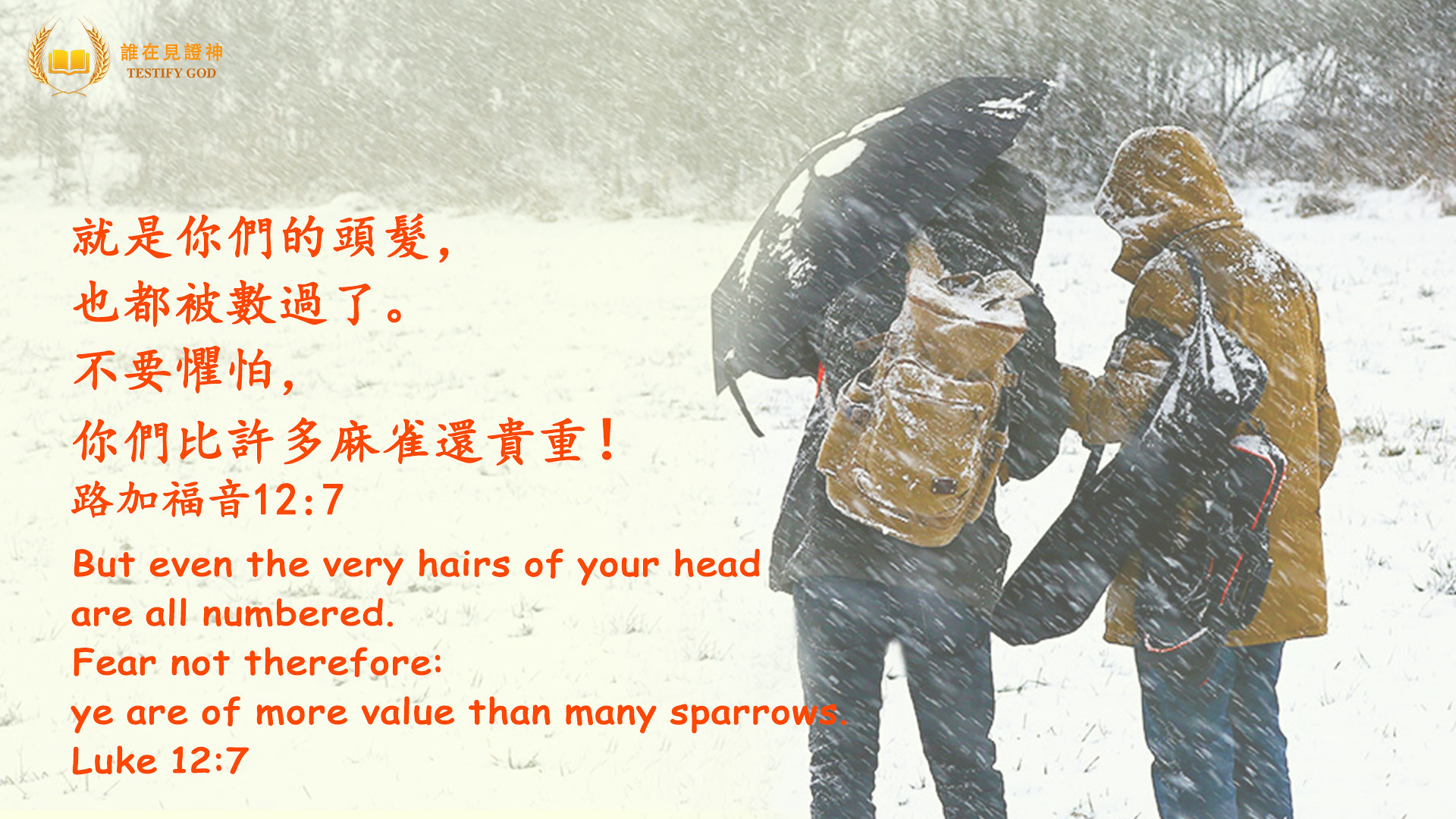The image depicts a scene during a heavy snowstorm set against a backdrop of dense, brown woods, where the snow has obscured much of the background, creating a white, snowy blur. In the right part of the picture, you can see the backs of two young people dressed for harsh weather. The person on the left is wearing a hooded brown coat, jeans, and has black bags with her, while the individual next to her, dressed in black, is shielding themselves with a black and white umbrella and has a brown backpack. Both have their hoods up to protect against the snow. The image includes text from an Asian Christian website, featuring Asian characters, and a Bible verse translated beneath: "But even the very hairs of your head are all numbered. Fear not therefore; ye are of more value than many sparrows." This verse, Luke 12:7, is prominently printed in red, with additional English text reading "Testify God." The snow is falling intensely, with daylight casting a subtle glow from the left side, illuminating the scene.